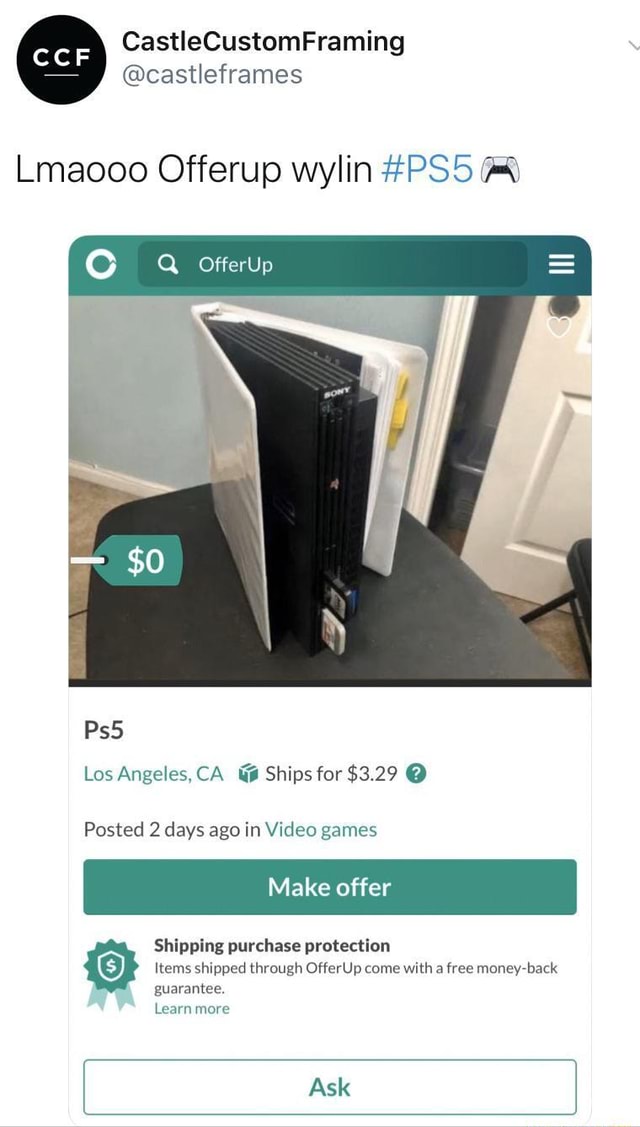Profile Picture: Black background with the white initials "CCF," underlined in white.

Username: @castlecustomframing (Castle Frames)

Caption: "LMAOOO, offer up #PS5 🎮"

Image Content Description:
- App Displayed: OfferUp
- Featured Item: PlayStation 5 (PS5)
- Description: A white PS5 console on a sleek, black table.
- Pricing Information: Listed for $0, displayed on a green price tag.
- Location: Los Angeles, CA
- Shipping Fee: $3.29
- Time Posted: 2 days ago
- Category: Video Games
- Action Button: A green "Make Offer" button
- Shipping Protection: Items shipped through OfferUp come with a free money-back guarantee.
- Additional Information: A "Learn More" link also highlighted in green.
- Inquiry Option: An "Ask" button, set in a white rectangle outlined in green with the text in green.

Overall, this OfferUp listing humorously showcases a PS5 offered for free, accompanied by the seller's playful caption and key details about the listing.